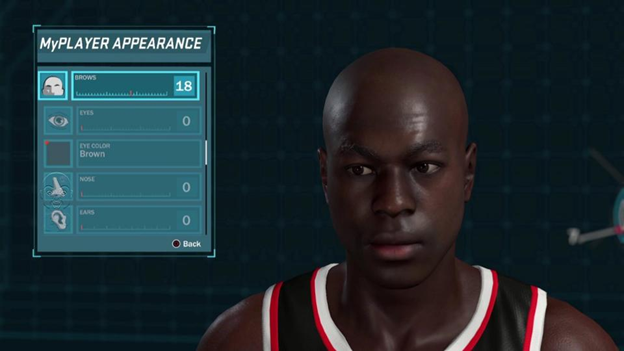Screenshot of a basketball video game showcasing the 'My Player Appearance' menu. The scene features a profile view of a basketball character with a black and bald head, dressed in a sleek black jersey adorned with red and white pinstripes. Against a dark background, the character is gazing off-screen to the right, not directly engaging with the viewer. To the left, a prominent blue dialog box is displayed, listing five user entries within the 'My Player Appearance' section. Although the text beside each entry is illegible, this menu likely offers various customization options for the player's avatar. The overall ambiance is both intense and focused, reflecting the immersive experience of the game.